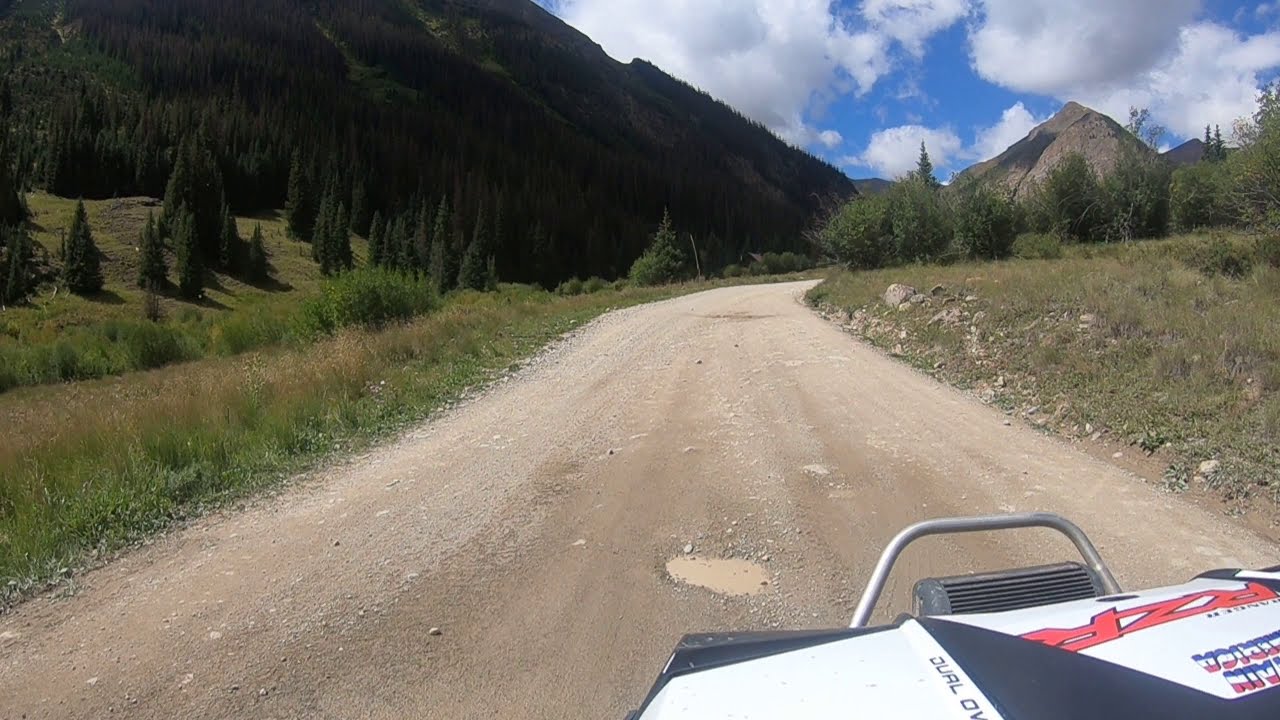The image is a detailed, color landscape photograph capturing a rugged dirt road that winds and narrows into the distance, eventually curving around a bend. The road is flanked on both sides by tall grasses, some green, some rocky, and others in shades of brownish-green. In the bottom right foreground, the partially visible hood of a moving vehicle, which appears to be a white and black car with "RZR" lettering, indicates the viewer's vantage point. This car is heading forward along the road. To the left of the road, the landscape features low trees, high bushes, and a hillside that rises into a mountainous area covered in tall, dark green pointed trees. In the background, the mountains ascend sharply, occupying the top left corner and middle upper part of the image, with a single pointed gray mountain visible in the top right distance. The sky is filled with clear, non-threatening clouds, allowing some sunshine to filter through, giving the scene a dynamic and exploratory feel in a lush, mountainous terrain.